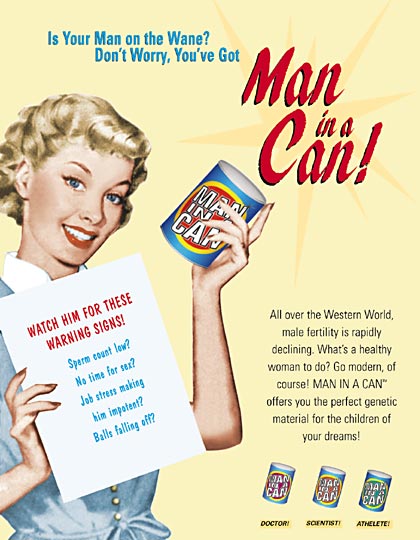The image portrays a tongue-in-cheek advertisement styled in a classic 1940s-1950s aesthetic. At the center of the scene is a woman with blonde hair and blue eyes, dressed in a retro house dress, holding a vibrant blue can labeled "Man in a Can" in striking red and yellow colors. The ad's bold headline reads, "Is your man on the wane? Don't worry, you've got Man in a Can," with "Man in a Can" emphasized in large red cursive font, while the accompanying text appears in a smaller blue print.

The image humorously outlines supposed warning signs to watch for in a man, including "sperm count low," "no time for sex," "job stress making him impotent," and "balls falling off." The satirical message states, "All over the Western world male fertility is rapidly declining. What's a healthy woman to do? Go modern, of course! Man in a Can offers you the perfect genetic material for the children of your dreams."

At the bottom of the advertisement, three cans are displayed, each labeled with a different ideal man's role: Doctor, Scientist, and Athlete. The overall design uses a combination of red, blue, and yellow colors, evoking the nostalgic feel of mid-20th-century print advertising while delivering its humorous and ironic message.